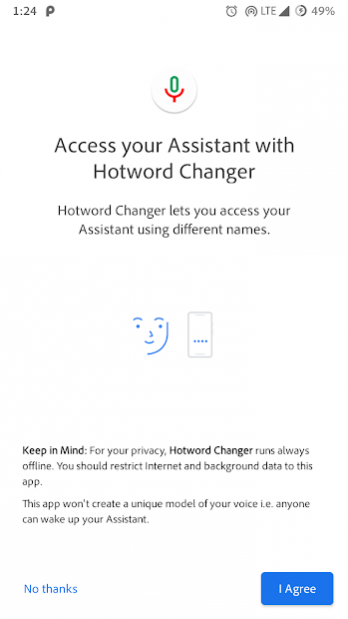The screenshot displays a smartphone interface on a white background. At the top, the status bar shows the time as 1:24, accompanied by an alarm clock icon, full signal bars, and a battery level at 49%. Below the status bar, the interface features a circular icon resembling a microphone in green and red. Underneath this icon, black text reads: "Access your assistant with Hot Word Changer. Hot Word Changer lets you access your assistant using different names."

Further down, there is a blue, stylized half-face with a smartphone illustration. Beneath this illustration, additional text advises: "Keep in mind for your privacy, Hot Word Changer runs always offline. You should restrict internet and background data to this app. This app won't create a unique model of your voice but can wake up your assistant."

At the bottom of the screen, the interface offers two options. On the left, in blue text, it says "No Thanks." On the right, a blue rectangular button with white text in the center reads "I Agree."